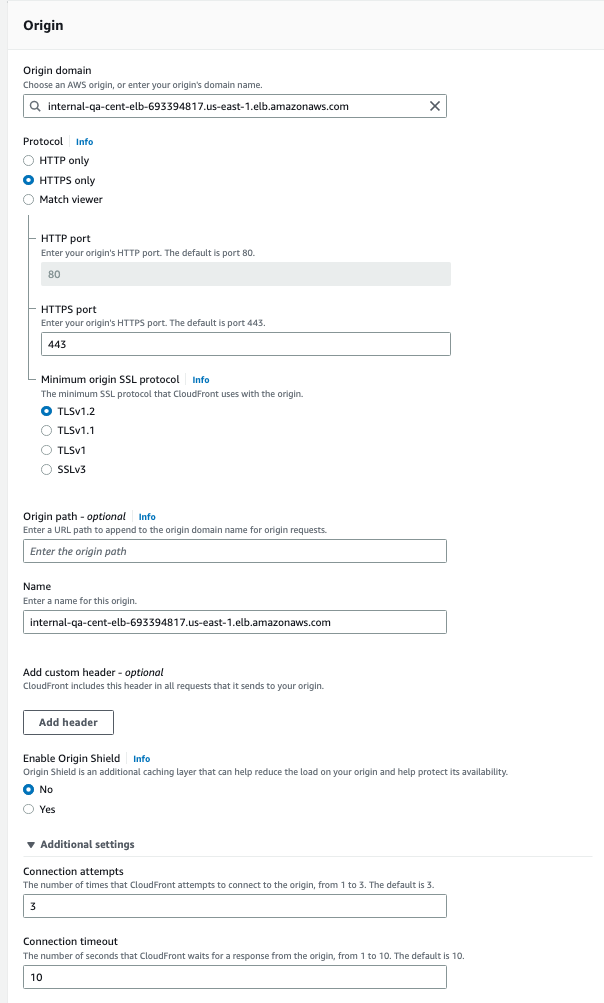The image depicts a configuration page for setting up an origin in AWS CloudFront. The interface appears to be either a screenshot of a computer display or a mobile device screen.

At the top, a light gray border banner reads "Origin," followed by directions to choose an AWS origin or input an origin domain name. Below it, a search bar allows users to enter the domain name.

Next, there's a list of protocol options: HTTP only, HTTPS only, or Match Viewer, with HTTPS only selected, indicated by a blue dot. Following this, instructions to enter the HTTP port with the default set to 80 are displayed, with the number 80 in a gray box underneath.

Below are details for entering the HTTPS port, with the default set to port 443, shown in a white text box with 443 already filled in. The section continues with the minimum origin SSL protocol, indicating the minimum SSL protocol that CloudFront will use with the origin. Next to this, a blue "info" button is present. The TLSv1.2 option is selected by a blue bullet point.

Further options include TLSv1.1, TLSv1, and SSLv3. The form also features an "Origin Path" field, marked as optional, with an accompanying blue "info" icon. Users are advised to enter a URL path to append to the origin domain name for requests, with a white text box below to input the origin path.

The section continues with a "Name" field to enter a name for the origin, followed by the name of the website. An "Add Custom Header" option is available, indicating that CloudFront will include this header in all origin requests. This is followed by an "Add Header" feature inside a white bordered box.

Lastly, the option to "Enable Origin Shield" is presented alongside a blue "info" button. This advises that Origin Shield is an additional caching layer that can reduce the load on the origin and protect its availability, with "No" being selected.

The caption concludes with additional settings including "Connection Attempts," with the number of times CloudFront will attempt to connect to the origin (ranging from 1 to 3, default set to 3) and "Connection Timeout," detailing the number of seconds CloudFront will wait for a response from the origin (ranging from 1 to 10, default set to 10). The respective text boxes display the default values of 3 and 10.